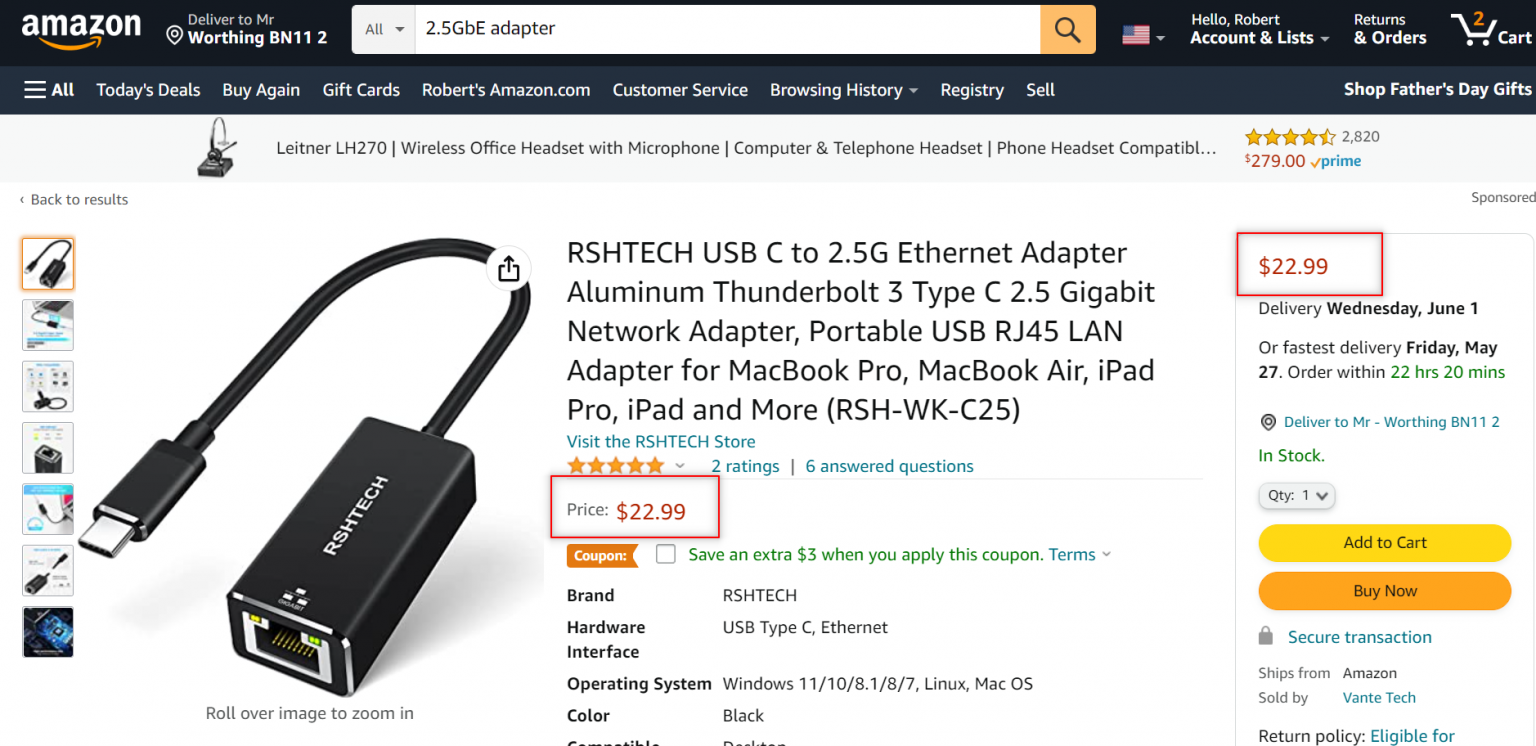This image showcases an Amazon product listing for a portable, high-speed 2.5 gigabit network adapter. The device, designed for connectivity through USB Type-C and Ethernet, is compatible with an array of devices including MacBook Pro, MacBook Air, iPad Pro, and more. It also supports various operating systems like Windows 11, 10, 8.1, 8, 7, Linux, and macOS.

The adapter, branded by RSH Tech, features a sleek black design with "RSH Tech" printed in white text. It's currently priced at $22.99, with an option to save $3 via a coupon. While it offers fast delivery by May 27th, standard shipping date is estimated around June 1st.

Sold by Vantay Tech and addressed to a customer possibly named Mr. Worthingby11, the product images can be seen on the left side, providing additional visual details. Despite having high ratings, the product has been reviewed by only two customers, indicating a relatively new listing.

The listing emphasizes the adapter's portability and versatility, making it a convenient accessory for users requiring a reliable network connection in various environments.